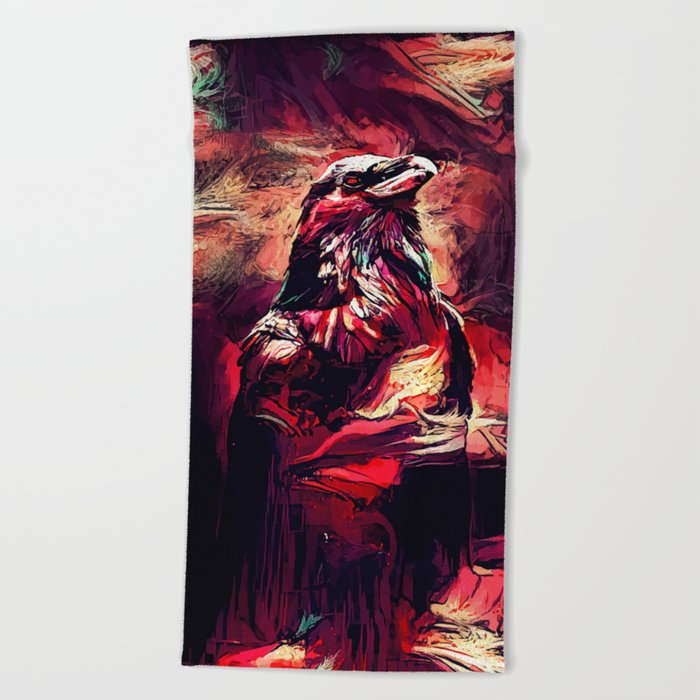The image depicts a regal eagle or perhaps a hawk, facing to the right, its red eyes adding a touch of menace. The bird is adorned in feathers that blend red, black, and purple hues, interspersed with splashes of green and gold for contrast. The background features a mix of reds and blacks, with some hints of orange and yellow, contributing to the overall dark and mysterious atmosphere. The artwork, which could be an oil painting or digital art, is presented on a vertically hung canvas, reminiscent of a movie poster. The setting behind the bird appears to be an abstract interpretation of a cave wall with swirling patterns and crevices. The bird's neck feathers show highlights of mauves, whites, and blues, while the lower part of the image seems to melt into a mix of flowing colors, giving the piece a somewhat surreal quality. The entire composition is highly detailed, revealing individual brush strokes, particularly around the wings and chest, creating an almost flowing effect that blends into the predominantly red background.